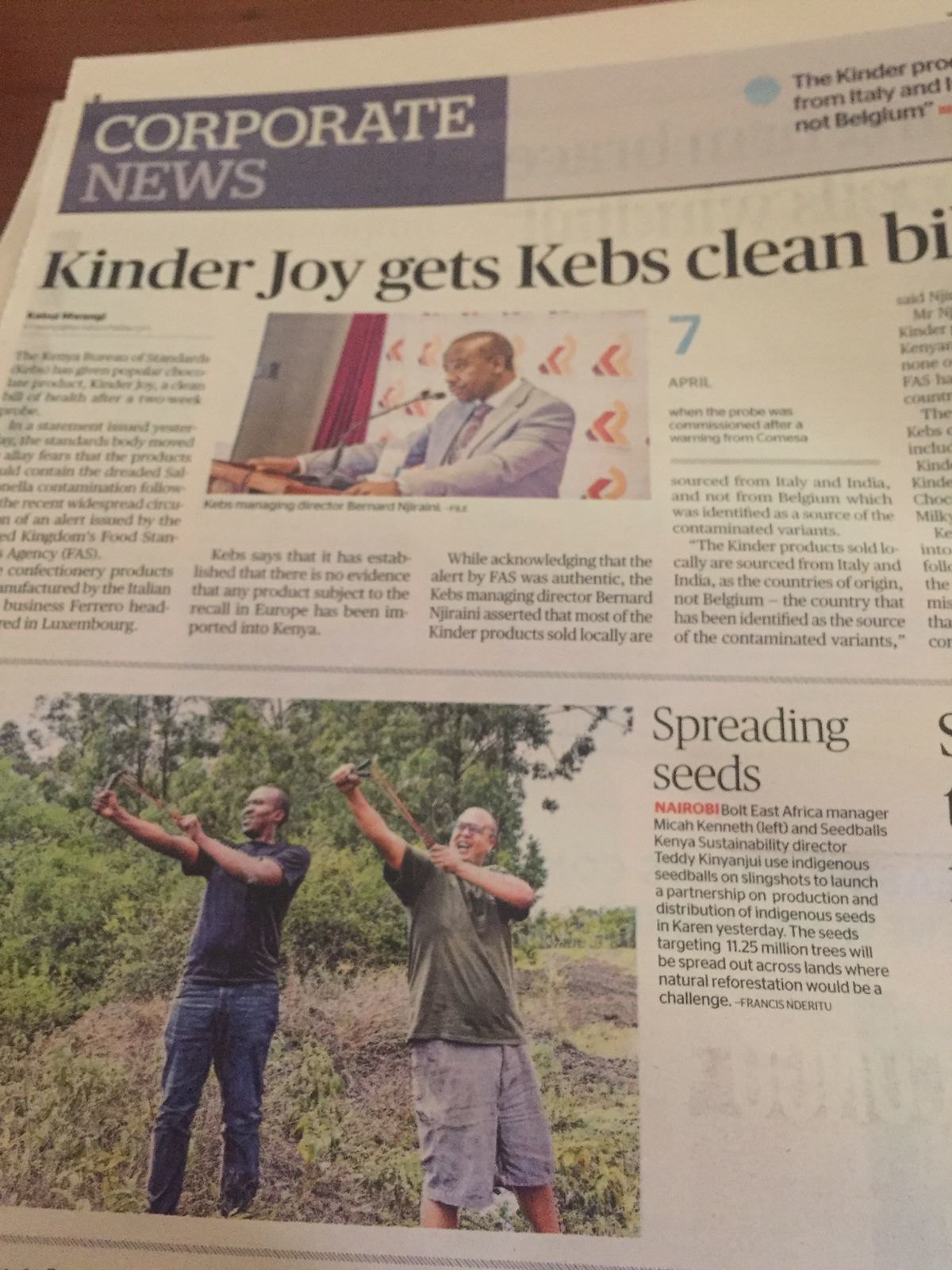The image shows a detailed layout of a newspaper page titled "Corporate News" in prominent white letters against a blue rectangular background in the top left corner. The newspaper features two main articles. The first article, whose title is partly visible as "Kinder Joy Gets Kebbs Clean, B.I.," is accompanied by a picture of a man in a gray business suit speaking at a podium with a microphone. This image sits against a white wall featuring an arrow pattern. The second article, titled "Spreading Seeds," includes a photograph of two men—one African American wearing a blue t-shirt and blue jeans, and the other a white man dressed in a green shirt and cargo shorts—engaging in an activity resembling rubber band archery in a natural setting with many trees in the background. The articles are separated by a horizontal gray line, and each article is followed by several rows of print, some of which extend beyond the visible edges of the image.